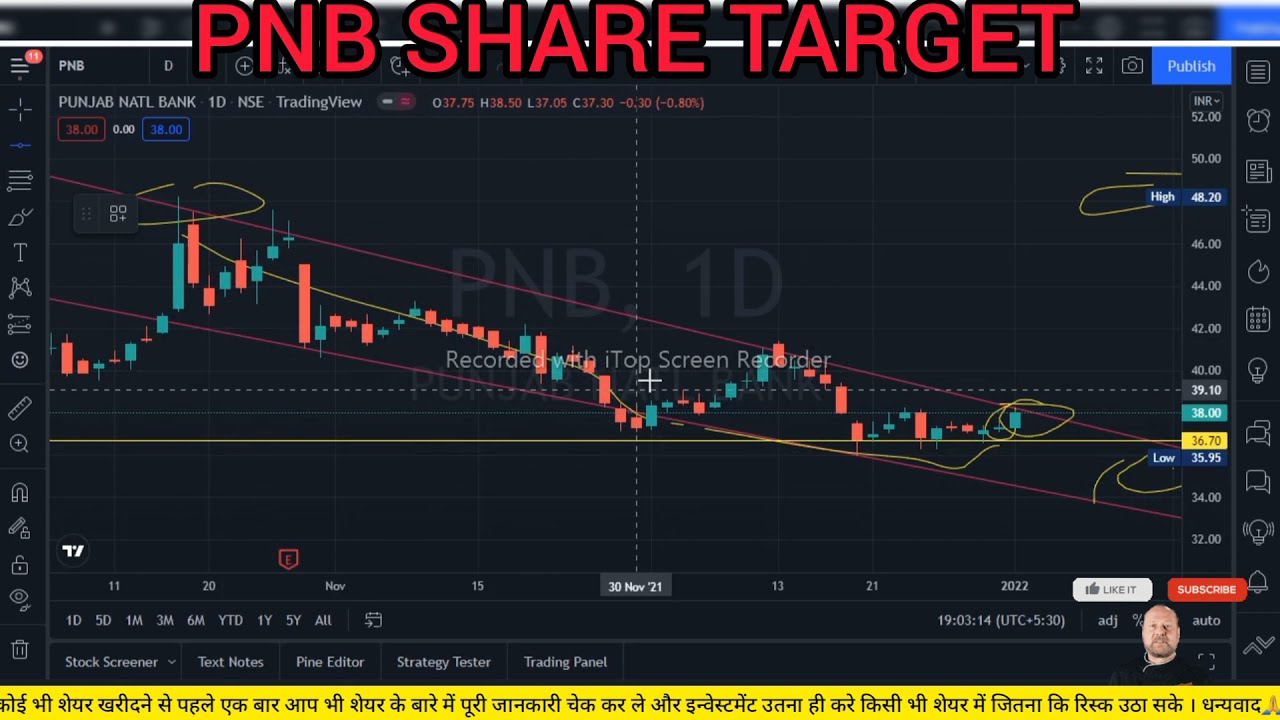The image depicts a screenshot of a financial market graph, likely related to stock market trends. The background is predominantly black, with grid lines and text in a language resembling Sanskrit or a Middle Eastern script, which is not readable. At the top of the image, bold red text states "P&B Share Target," and immediately below it, in smaller white letters, it reads "Punjab National Bank."

The graph itself features red and green trend lines laid out over the grid pattern, indicating some market movements. Additionally, there are numerous icons on both the left and right sides of the screen: a T for text, a smiley face, a ruler, a magnet, a pencil, a lock, an eye, a trash can, and a magnifying glass among others. These icons suggest that the image is a screen capture from some stock analysis or financial charting software.

Across the bottom of the image, timeframes such as "1 day," "5 days," "1 month," "3 months," "6 months," "Year to Date," "1 year," "5 years," and "All Time" are listed, reinforcing the stock market context. There's a notable yellow bar at the very bottom with black text, possibly in Arabic or another unfamiliar script. 

The image also features pink and blue vertical cylinders representing different data points, closely aligned with the chart's fluctuating lines. Additional details include small, unreadable white text in various sections and a faint, transparent overlay of the text "P&V, 1D" over the graph area. Lastly, there's a small image of a bald-headed, white, American man with facial hair in the bottom right corner, likely offering instructions or commentary on using the financial software depicted.